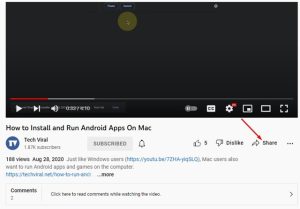Screenshot Analysis: YouTube Video Interface with Specific Details

The screenshot showcases a YouTube video view where the video titled "How to Install and Run Android Apps on Mac" is paused at the very beginning. The video has just started as indicated by the red progress bar, which barely extends past the volume button, suggesting minimal playback progress. The loading status, shown by the gray part of the progress bar, does not surpass the timestamp area.

In the video player control area at the bottom, several icons and indicators are visible:
- A white play button triangle pointing to the right.
- A fast-forward triangle icon with a vertical line at its tip next to the play button.
- A volume icon positioned further to the right.

The current timestamp appears to be "0:32/9:10," though it is slightly pixelated, making it challenging to read.

Above the timestamp, a light gray rectangular area displays the video title in bold black text: "How to Install and Run Android Apps on Mac." Directly below this, on the left, sits the user (channel) icon of the video uploader. The channel icon is a blue circle featuring a slanted white window with a black silhouette in the middle.

To the right of the user icon, the channel name "Tech Viral" is displayed in black text, with the subscriber count written below it in light gray small font, reading "1.87k subscribers."

This thorough description effectively captures the various elements of the YouTube video interface and the specifics presented in the screenshot.